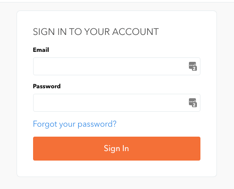The image depicts a sign-in box, which could be from either a website or a mobile site. The box has a nearly square shape with a light gray border and a white background. At the top of the box, there is dark gray text that reads, "Sign in to your account." Below this, there is an entry field labeled "Email" in black text, meant for users to input their email addresses. Following the email entry field is another one labeled "Password," also in black text, for users to enter their passwords. Above the sign-in button, there is a blue link that reads, "Forgot your password?" The sign-in button itself is orange with white text that says "Sign In."